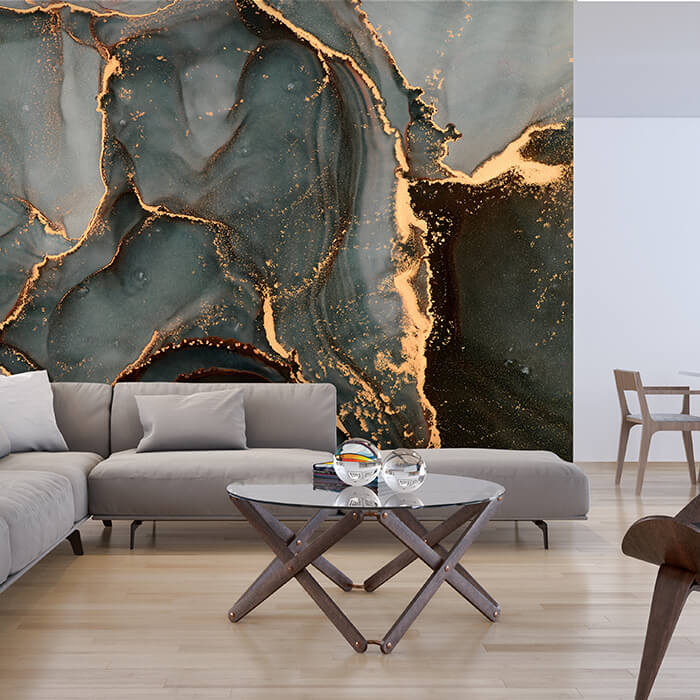This photograph, taken indoors, showcases a meticulously designed living room centered around a modernistic glass coffee table with distinct X-shaped wooden legs. On the table, two glass orbs sit side by side, with the larger orb positioned to the left. A book or similar item rests behind these orbs. Dominating the seating area is a sleek sectional sofa in a shade of gray, complemented by gray throw pillows. Behind the sofa, a dramatic mural spans the entire wall, illustrating a rocky landscape with rugged, wrinkly textures. This dynamic artwork features contrasting bright yellow lines that evoke the image of light breaking through the grayscale landscape, adding an eye-catching, vibrant touch to the room. The right side of the mural is bordered by a wooden chair, while another wooden chair or stool is visible in the bottom right corner of the photograph. The room's flooring is composed of elegant wood planks, enhancing the overall sophisticated ambiance of the space.